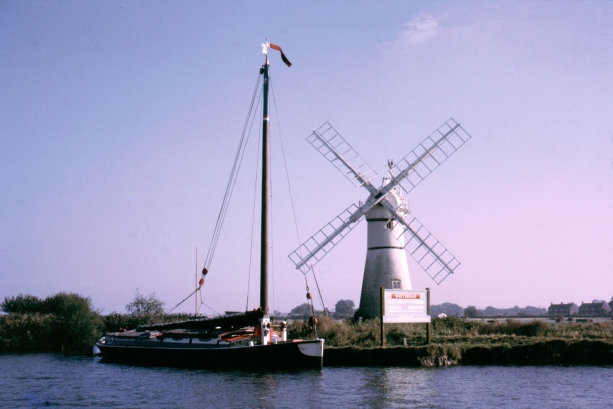The photograph captures a serene blue-tinted landscape at either dusk or dawn, enhancing the tranquil atmosphere with a purple gradient sky and light scattered clouds. In the reflective dark blue water of the foreground, a small sailboat rests with its sail down, though the mast and a red and black flag are visible. This sailboat, with its intricate strings and ropes, sits near the left side of the image. Behind it, slightly to the right, stands an old-fashioned white windmill with a thick grayish-white cylindrical base and see-through metal blades. The windmill is positioned on a green, unkempt grassy landmass that extends to the horizon. A sign with large white writing over a red background, mostly white, is posted near the windmill on the right. Adding to the complexity of the scene, a hint of a distant town can be seen on the far right, bordering the softly illuminated waterscape.